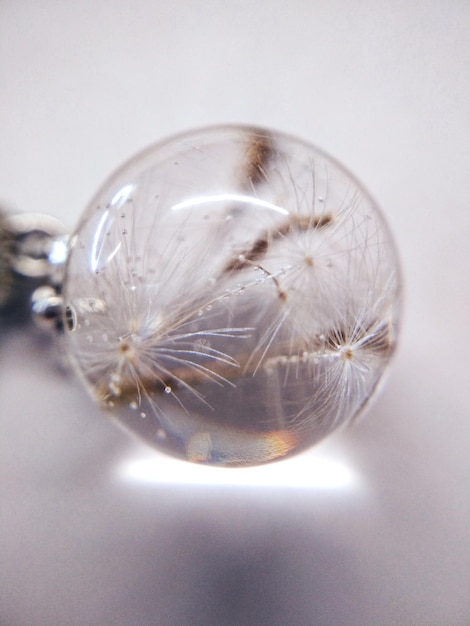The photograph depicts a crystal-clear spherical orb, possibly the top of a scepter, situated against a whitish-gray background. Illuminated by natural light, the orb, which might be glass or crystal, showcases intricate details inside. Encased within it are delicate, feather-like structures reminiscent of dandelion seeds, each featuring a brown spot at its center with fine tentacle-like extensions. These internal elements resemble spider webs or twigs, possibly even insect-like forms, but most distinctly dandelion spores. The sphere is mounted on a metallic fixture, visible through hints of silver and black at its base. The light enhances the orb's clarity, making the inner contents stand out as the primary focal point, surrounded by subtle reflections.